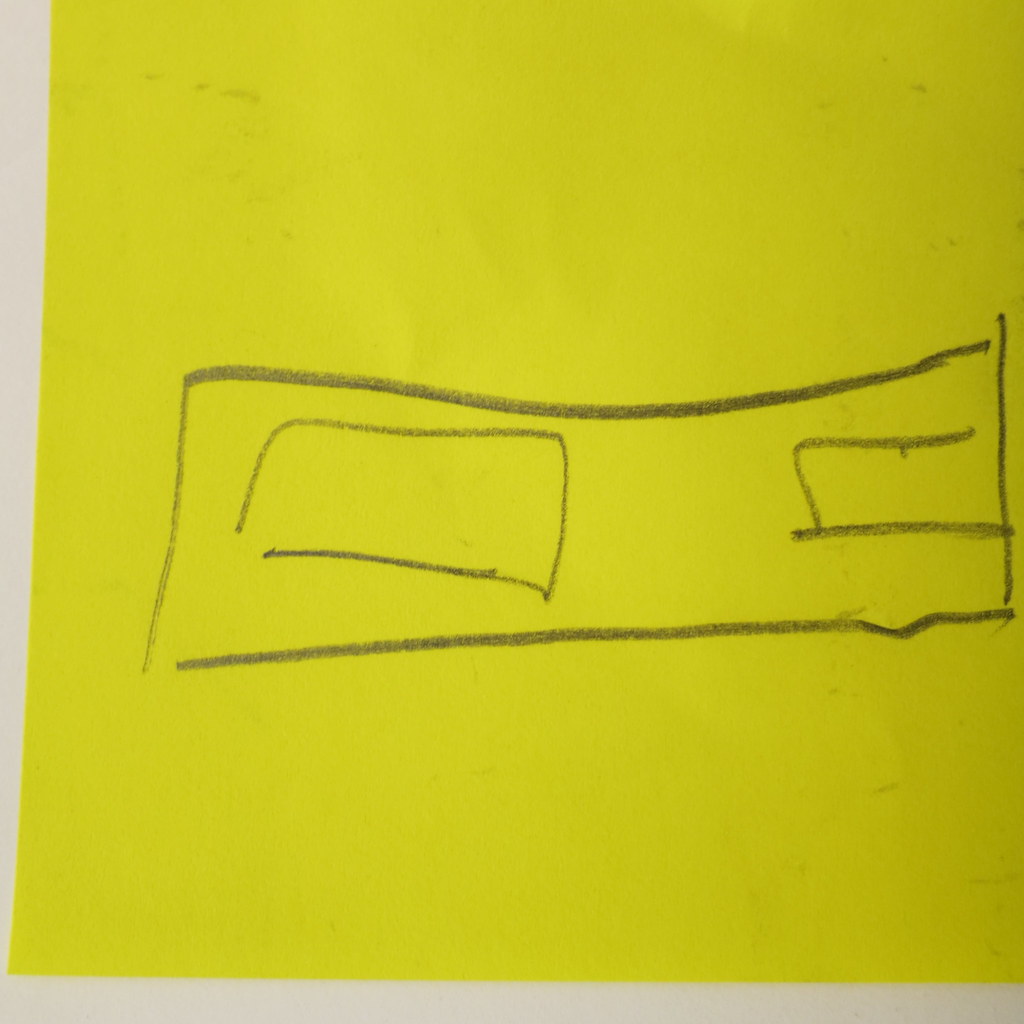A close-up image showcases a sticky note that fills most of the frame, with slight white margins visible on the left and bottom edges. The focus on the sticky note enlarges its appearance. Dominating the center of the note is a roughly sketched large black rectangle, drawn with what appears to be a crayon or similar utensil. Inside this large rectangle are two smaller rectangles: the one on the left is larger and more complete than the smaller, less defined one on the right. The lines of these rectangles are irregular and chaotic, indicating a hasty drawing process. Smudges are particularly noticeable in the bottom right corner of the large rectangle. The drawing's imperfect lines and smudged appearance add a layer of texture and intrigue to the otherwise simple composition.